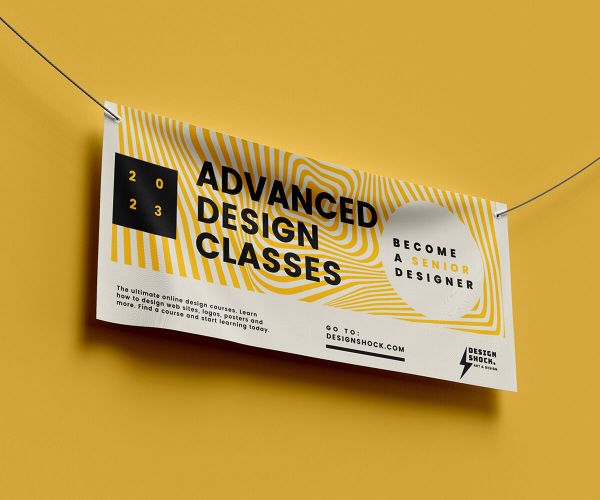The photograph shows a rectangular banner hanging indoors against a dark golden butter yellow background. The banner is approximately two inches wide and one inch high, suspended by a black string that starts from just below the upper left-hand corner, travels diagonally downward to meet the banner, and then continues diagonally upward towards the center right of the image. The banner itself features a detailed design with a predominantly white background. 

At the top of the banner, yellow stripes converge into a spiraling circle, creating a dynamic visual effect. To the left, there is a black square with gold lettering displaying "2023." Bold black text across the middle of the banner reads "Advanced Design Classes." On the right side, another key detail includes a white circle with black text saying "Become A," followed by the word "Senior" in gold, and beneath that, in black, "Designer."

Below this, the banner has a white-bordered section hosting three lines of black text explaining, "The ultimate online design courses. Learn how to design websites, logos, posters, and more. Find a course and start learning today." The text "Go to DesignShock.com" is prominently underlined in the center. Finally, towards the lower right, there is a black lightning bolt symbol next to the name "DesignShock."

Overall, the detailed banner presents a comprehensive advertisement for advanced design classes, promoting the DesignShock website as a resource for aspiring senior designers.